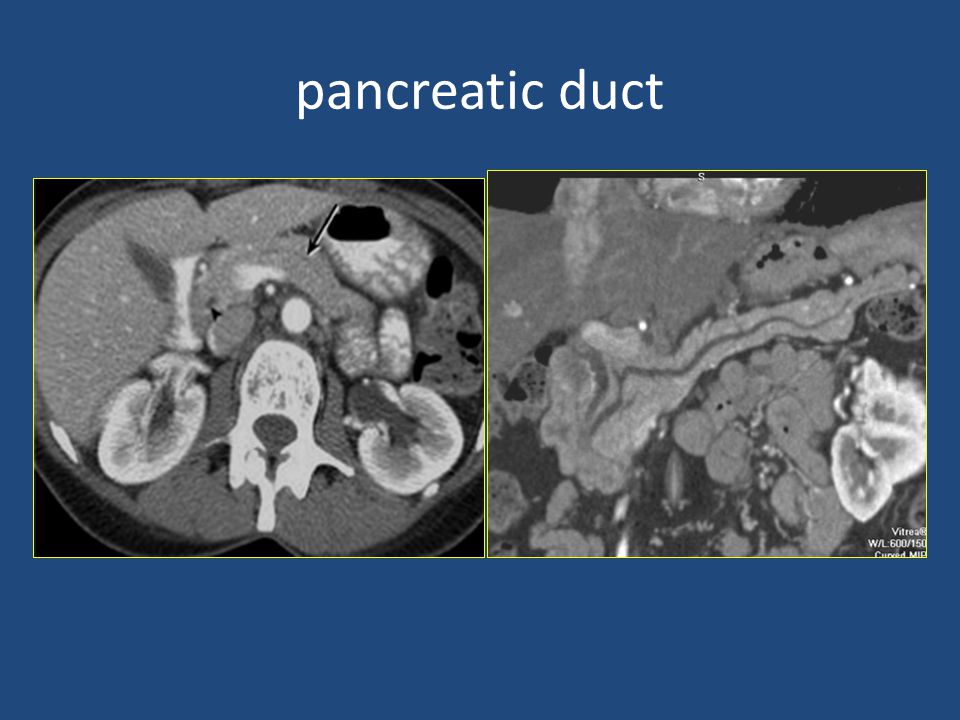This image appears to be an educational slide, likely from a medical journal or textbook. The slide features a blue rectangular background with white lowercase lettering at the top that reads "pancreatic duct." Below the title, there are two black-and-white photographs of the pancreatic duct positioned side by side. The photograph on the left provides an overview with an arrow specifically pointing to the pancreatic duct, while the photograph on the right appears to be a more detailed, dissected view revealing the internal structure of the duct. Both images may have been obtained using microscopic techniques or internal cameras, showcasing the pancreatic duct in varying shades of black, gray, and white. In the lower right-hand corner, the slide includes additional notations: "vitra W/L 600/150" and "curved VIP," suggesting technical details related to the imaging or presentation format.